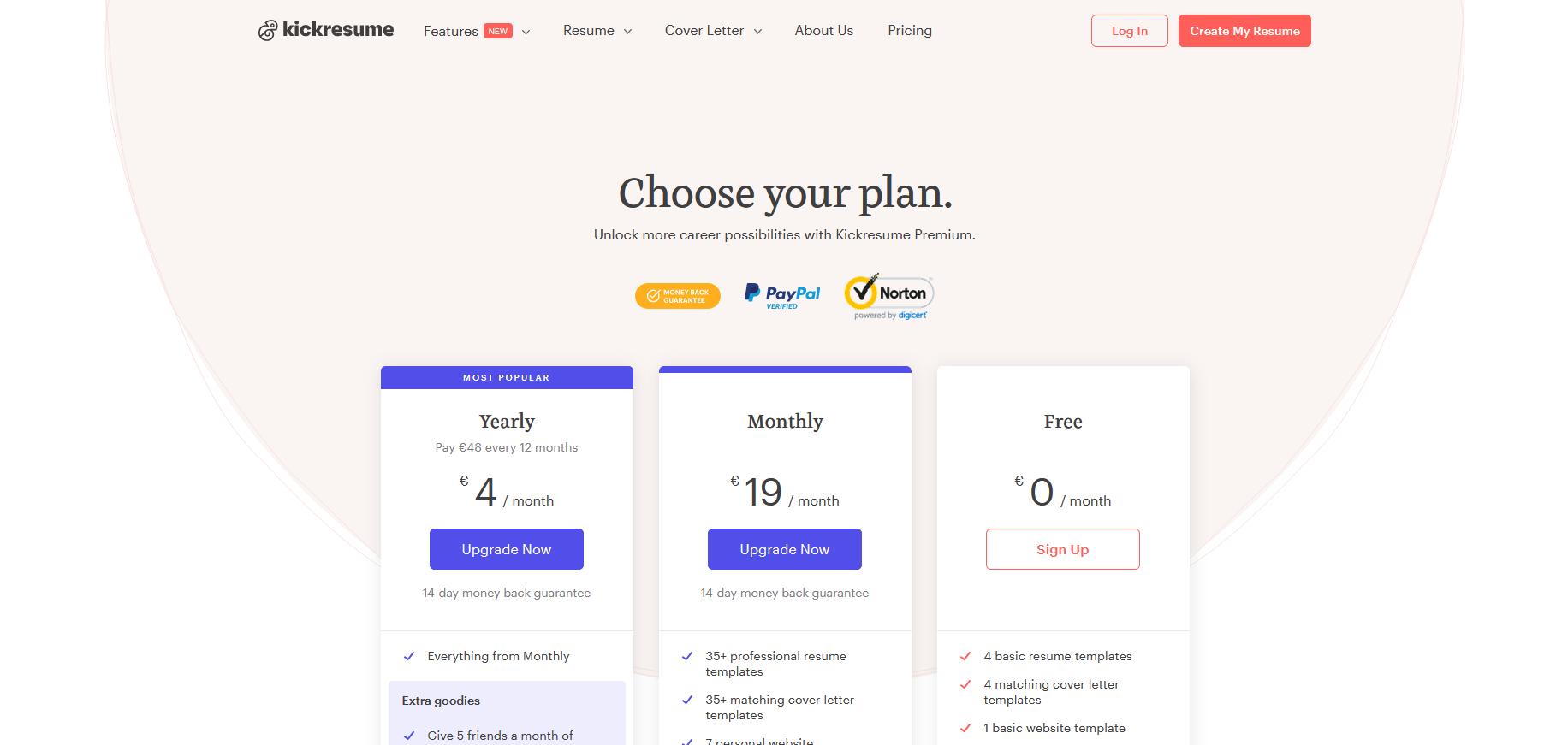The image appears to be the homepage of a business named Kick Resume. In the upper left-hand corner, the logo, which includes an outline of a snail-like creature, is displayed next to the company name "Kick Resume." The navigation bar spans from left to right and includes the following options: Features (with a drop-down menu), New (drop-down menu), Resume (drop-down menu), Cover Letter (drop-down menu), About Us (no drop-down menu), and Pricing (no drop-down menu). On the right side of the navigation bar, there is a "Login" link in red text, and a red button with white letters that reads "Create My Resume."

Below the navigation bar, a section invites users to "Choose Your Plan, Unlock More Career Possibilities with Kick Resume Premium." Beneath this, a yellow box highlights a "Money Back Guarantee," with verification badges for PayPal and Norton secured by DigiCert. 

The pricing plans are detailed in a comparative format labeled "Most Popular." The yearly subscription, marked as the most popular plan, is priced at £48 every 12 months (equivalent to £4 per month), featuring an "Upgrade now" option, and emphasizes a 14-day Money Back Guarantee. This plan includes full blue tick marks for features such as "35+ Professional Resume Templates," "35+ Matching Cover Letter Templates," and "7 Personal Websites," among others.

Beside the yearly plan, the monthly subscription is priced at £19 per month, also featuring an "Upgrade now" button in a blue color and a 14-day Money Back Guarantee. This plan also includes several features with blue tick marks similar to the yearly plan.

On the far right, the Free plan is displayed, indicated by a box outlined in red. It shows a "Sign Up" button in red text. The Free plan includes features marked with red ticks, such as "4 Basic Resume Templates," "4 Matching Cover Letter Templates," and "1 Basic Website Template."

Overall, there is no additional text or information provided in the image.